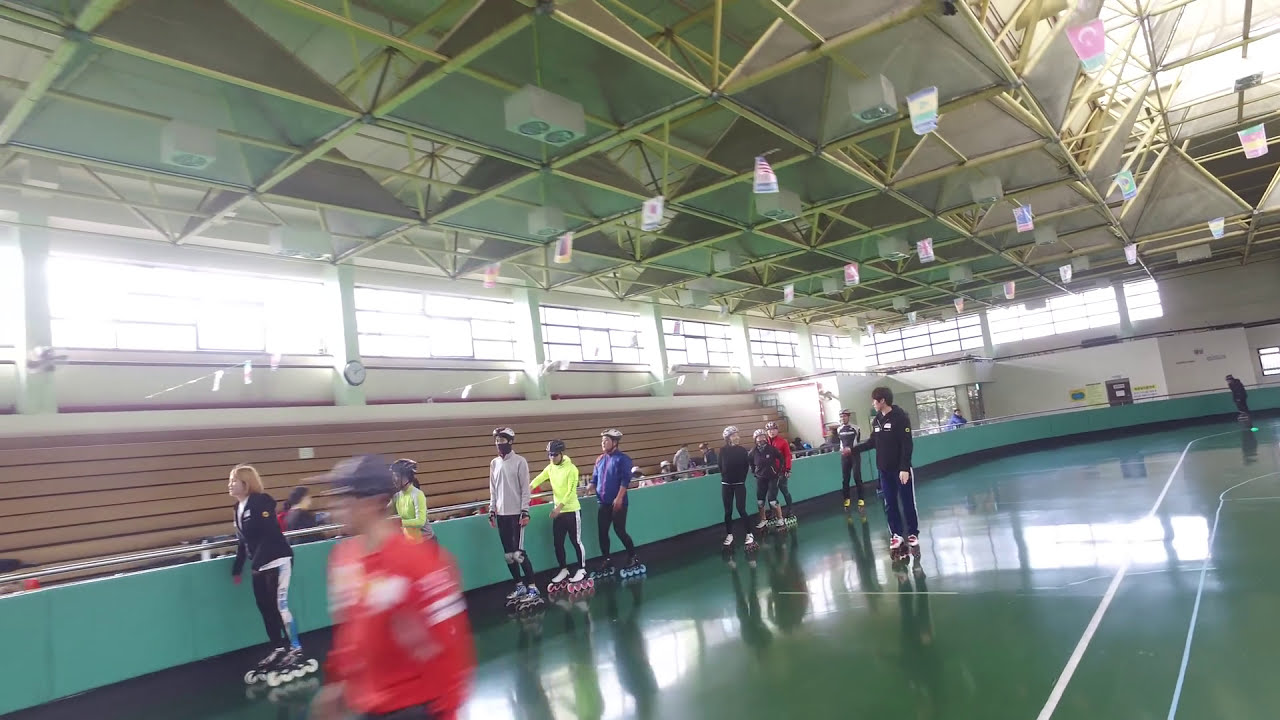In this vibrant scene, we are inside an indoor roller rink with a polished green floor and white striping designating skating areas on the lower right. The rink is encircled by a low aquamarine wall that curves from the left around to the lower right, leading up to rustic brown bleachers. Above, a grid ceiling featuring structural framework, fans, and bright lights, lets in an abundance of natural light through large rectangular windows on the left-hand side. These windows continue around, creating a well-lit, airy atmosphere. The rink is teeming with skaters gliding from right to left; some are in helmets, and others without, utilizing both inline skates and roller skates. They sport an assortment of colored clothing, mainly in long sleeves and long pants, with shades of purple, yellow, beige, and dark blue. A blurred skater in a reddish shirt and a purplish hat stands out on the bottom left. The scene conveys both the lively energy of the skaters and the multifunctional use of the venue, emphasizing the supportive walls where some beginners cling as they learn to skate.